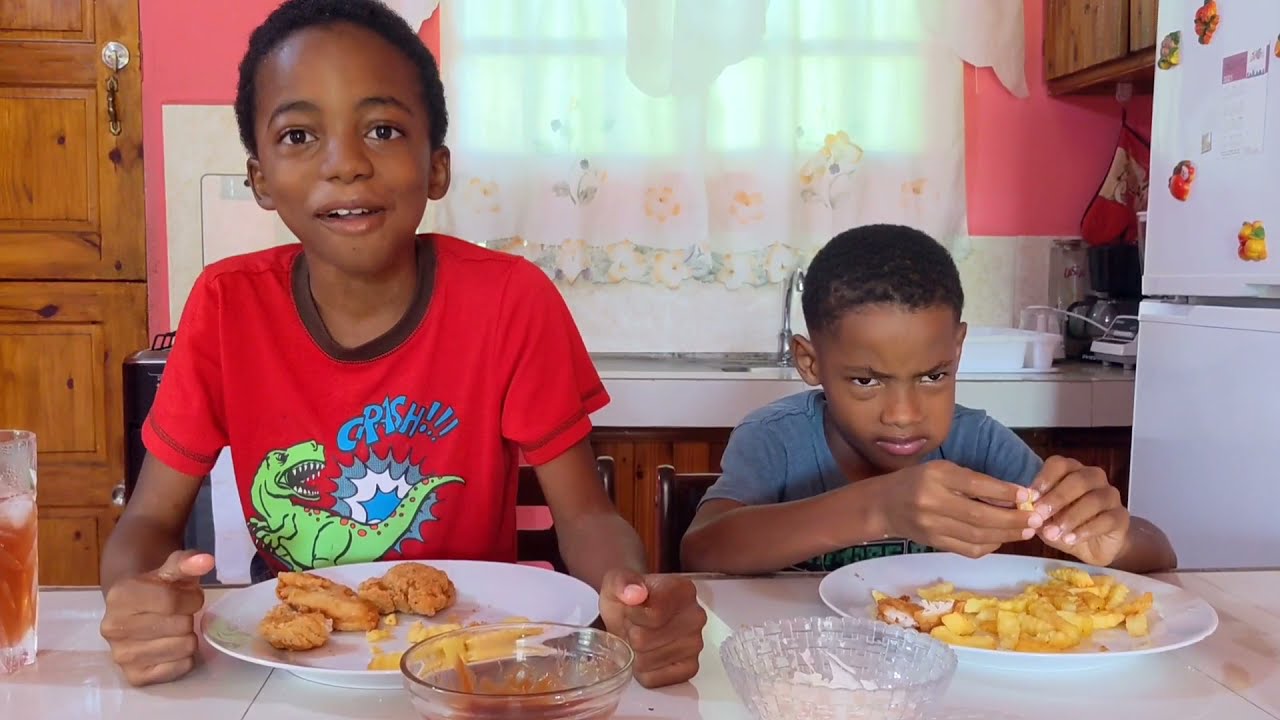The image captures a domestic scene in a kitchen where two young black boys are seated at a dining or kitchen table. Behind them, a refrigerator adorned with magnets stands to the right, while directly behind them are wooden cabinets, a silver sink, and a countertop. A window with a white curtain offers some natural light to the room, which features a mix of colors including red, green, blue, white, yellow, brown, black, gray, orange, and purple. The boy on the left wears a red shirt with a green Tyrannosaurus Rex graphic and "Crash" written in blue. He appears happy and sits up straight with his fists on the table. His plate is filled with chicken nuggets and French fries. The boy on the right, in a blue t-shirt, sports a grumpy expression and is slumped over, holding a piece of chicken in his hands above his plate, which has fewer chicken pieces and more fries. In front of them are clear glass bowls, one containing barbecue sauce and the other possibly ranch, as well as a cup that looks like iced tea. The boys' black chairs add to the cozy, everyday atmosphere of this kitchen meal setting.